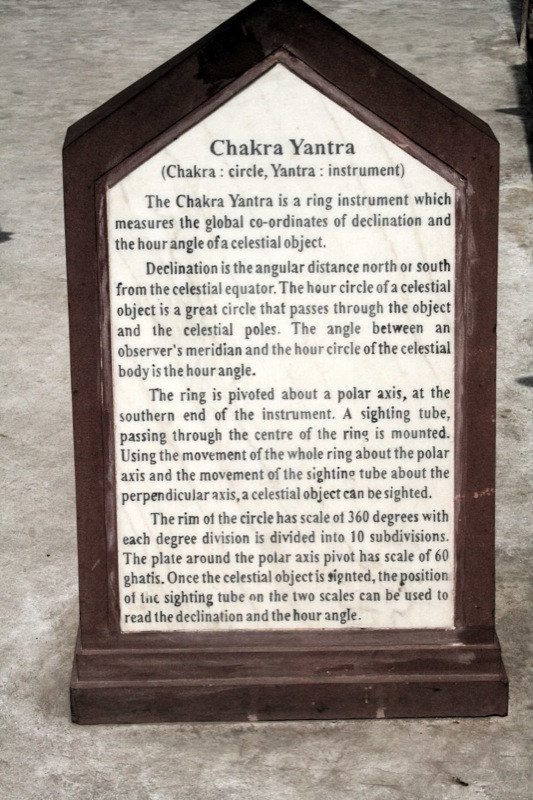This photograph depicts a vertically-oriented, five-sided wooden frame resembling the shape of a house, positioned against what appears to be an old cement or stone surface, possibly part of a road, parking lot, or indoor setting. The frame features a white background with black serif text. At the top peak of the frame, bold lettering reads "Chakra Yantra". Beneath this, in smaller text, parentheses clarify the term as "Chakra: Circle, Yantra: Instrument".

The text explains that the Chakra Yantra is a ring instrument used to measure the global coordinates of declination and the hour angle of celestial objects. Declination is defined as the angular distance north or south from the celestial equator. It further details that the hour circle of a celestial object is a great circle passing through both the object and the celestial poles. The hour angle is then described as the angle between an observer's meridian and this hour circle.

Additional paragraphs elaborate on the instrument's structure and functionality. The ring is pivoted about a polar axis at its southern end, with a sighting tube mounted through the ring's center. By manipulating the ring about the polar axis and adjusting the sighting tube along a perpendicular axis, one can target a celestial object. The rim of the ring is marked with a 360-degree scale, further divided into ten subdivisions, while a separate scale around the polar axis pivot features gradients of 60 divisions. Once the celestial object is sighted, the position of the sighting tube on these scales allows for the reading of its declination and hour angle.

The wooden frame appears to rest on a cement or stone pedestal, giving the presentation an academic or historical context.